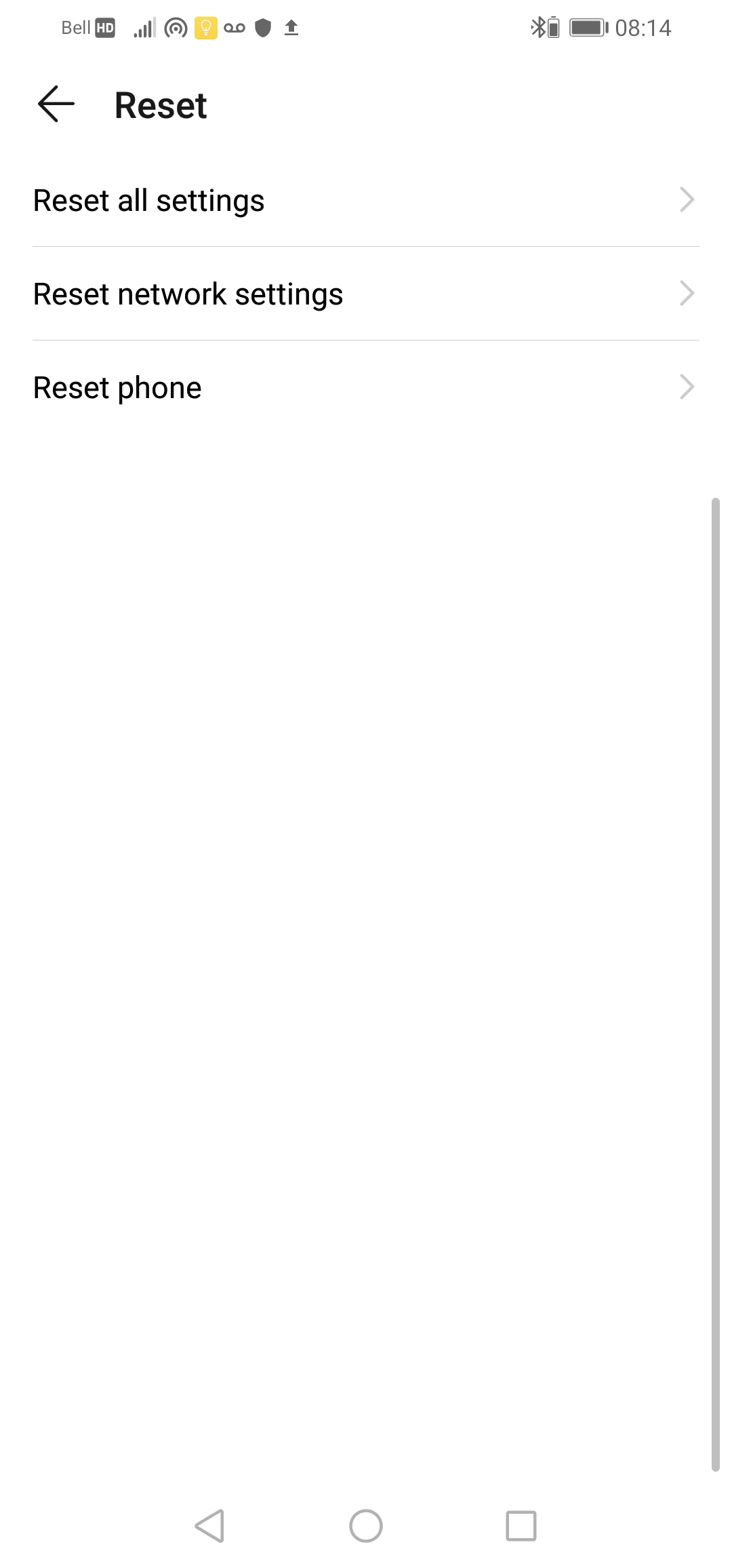Screenshot from an Android mobile device displaying a settings screen under reset options in light mode. The bottom of the screen features the standard navigation icons for Back, Home, and Tabs. The status bar on the top right indicates a full battery charge, Android version A14, and a Bluetooth icon next to another vertical battery icon possibly showing the Bluetooth device’s battery level. On the left side of the status bar, a series of icons are present, including a "Dell HD" icon, a signal strength icon with four out of five bars, and various other icons, one resembling a shield and another indicating a recent upload.

The primary content of the screenshot displays three reset options with switches to the right of each: "Reset all settings", "Reset network settings", and "Reset the phone." The page has a significant amount of white space, making it appear uncluttered and clearly showing that it’s configured in light mode.